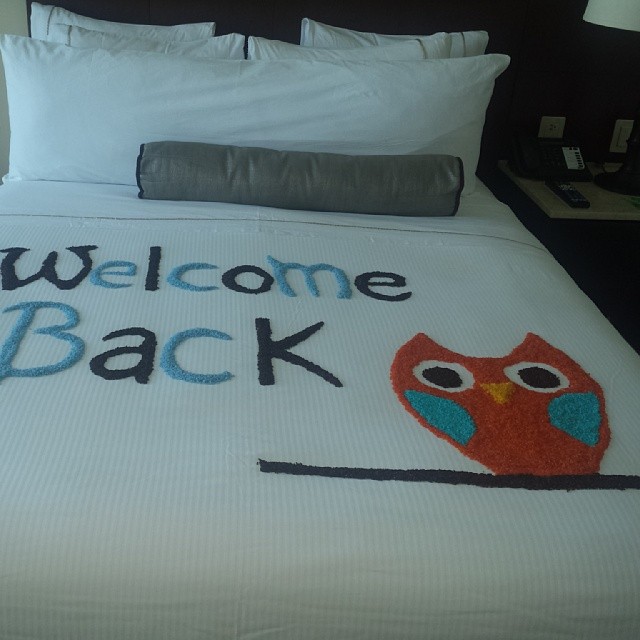In the image, a hotel bed occupies the majority of the dark bedroom, taking up around 90% of the picture. The bed is adorned with a white quilted bedspread that bears the stitched greeting “Welcome Back” in black and light blue letters. Below the welcoming text, a stylized red owl with black eyes, encircled by white, and blue feather highlights, perches on a brown or black line representing a branch. The bed features an arrangement of pillows, including a large long cylindrical gray foam roller pillow and several fluffy white pillows propped against the headboard. To the right of the bed, a marble-topped nightstand holds a remote control and a telephone with numerous buttons for different extensions—emphasizing the hotel room setting. The dim light barely reveals a phone jack and a wall jack near the nightstand.